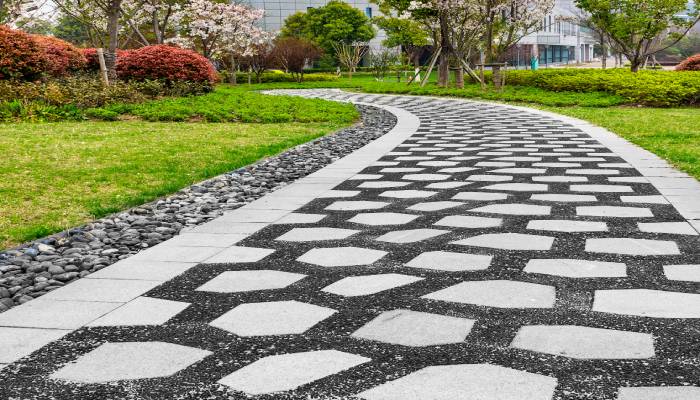The image captures a vibrant outdoor scene, seemingly located on the grounds of a hospital or commercial building. The photograph, taken on a clear sunny day, features a unique pathway that extends from the foreground and curves towards a large but partially visible building in the background, with numerous windows adorning its facade. This pathway is composed of wide stepping stones interspersed with black gravel, bordered by grey tiles and a smaller adjacent rock path. Flanking the walkway are patches of well-maintained grass and an array of colorful vegetation, including several trees with pink cherry blossoms, green trees, and shrubs adorned with red flowers. The image's low perspective emphasizes the intricately designed path and highlights the lush, vivid colors of the surrounding greenery.